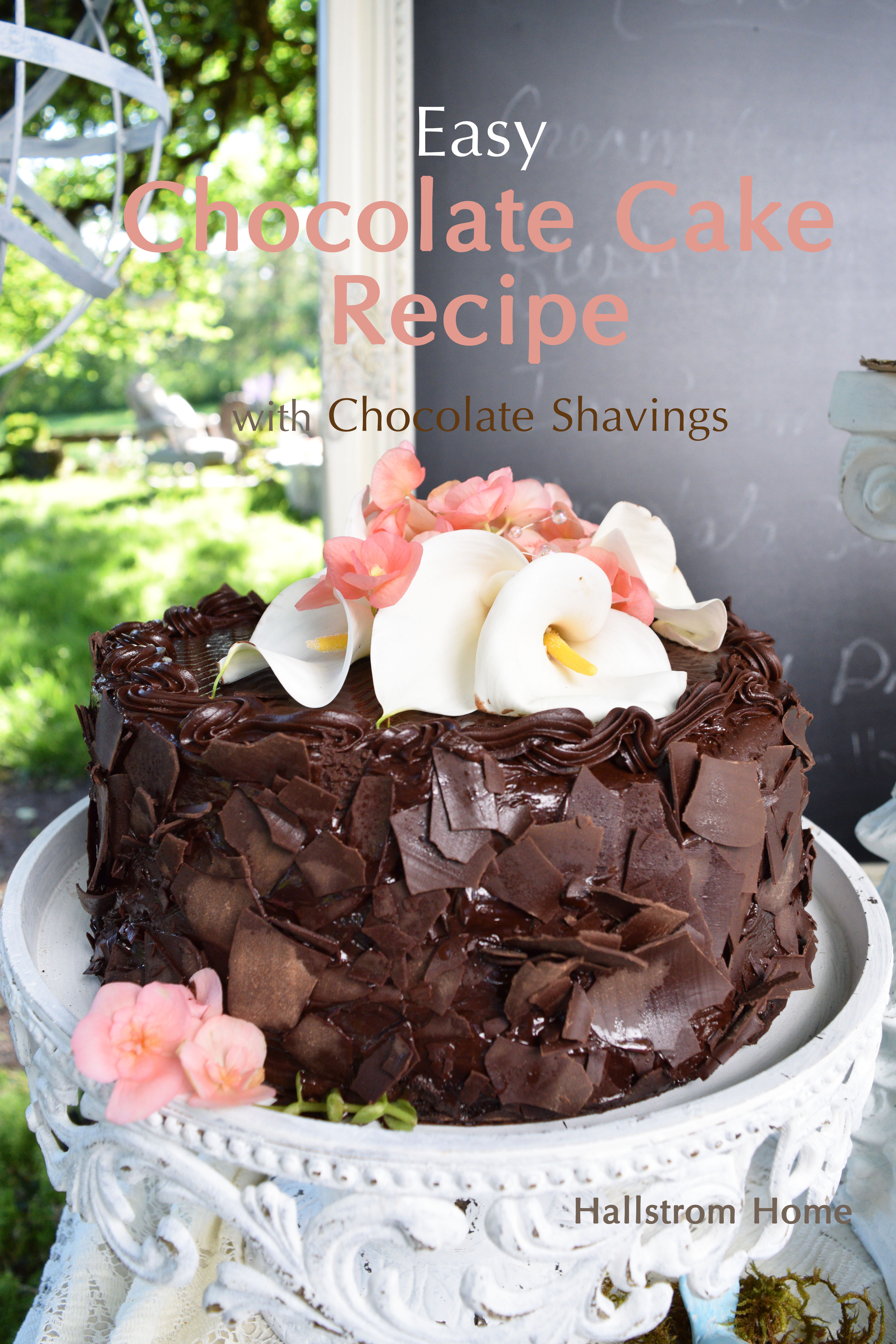The image depicts a beautifully decorated chocolate cake, entirely enrobed in rich chocolate frosting, with chocolate flakes or shavings adorning the sides. The top of the cake features the inscription "easy chocolate cake recipe with chocolate shavings," written in both white and pink text. Complementing the indulgent chocolate are large, realistic-looking white and pink flowers, likely real, with additional pink buds placed on the ornate white cake stand below the cake. This cake stand sits elegantly on a white lace tablecloth. The backdrop of the image includes a blurred, green outdoor scene, perhaps suggesting a garden or backyard setting, with a white piece hanging and some white chairs visible in the background. There's also a chalkboard with a white wood border, adding a rustic touch. At the bottom, the text "Hallstrom Home" is visible, hinting that this image might be the front of a cookbook or magazine.